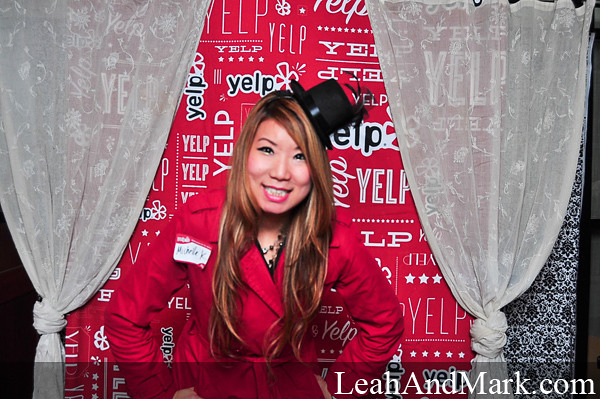In the image, an Asian woman with reddish-brown, mid-length hair stands smiling and leaning slightly forward in front of a red backdrop adorned with the word "Yelp" in various fonts, sizes, and orientations in both black and white text. She wears a red jacket and a small, lopsided black party top hat that appears too small for her head. Around her neck, she's adorned with various necklaces, and a name tag, though unreadable, is pinned on the left side of her chest. Her hands rest on her hips, adding a touch of playful confidence to her pose. White, sheer curtains tied into knots at the bottom frame the Yelp-themed backdrop on either side. Prominently displayed at the bottom right corner of the image is the semi-transparent white text "leahandmark.com."